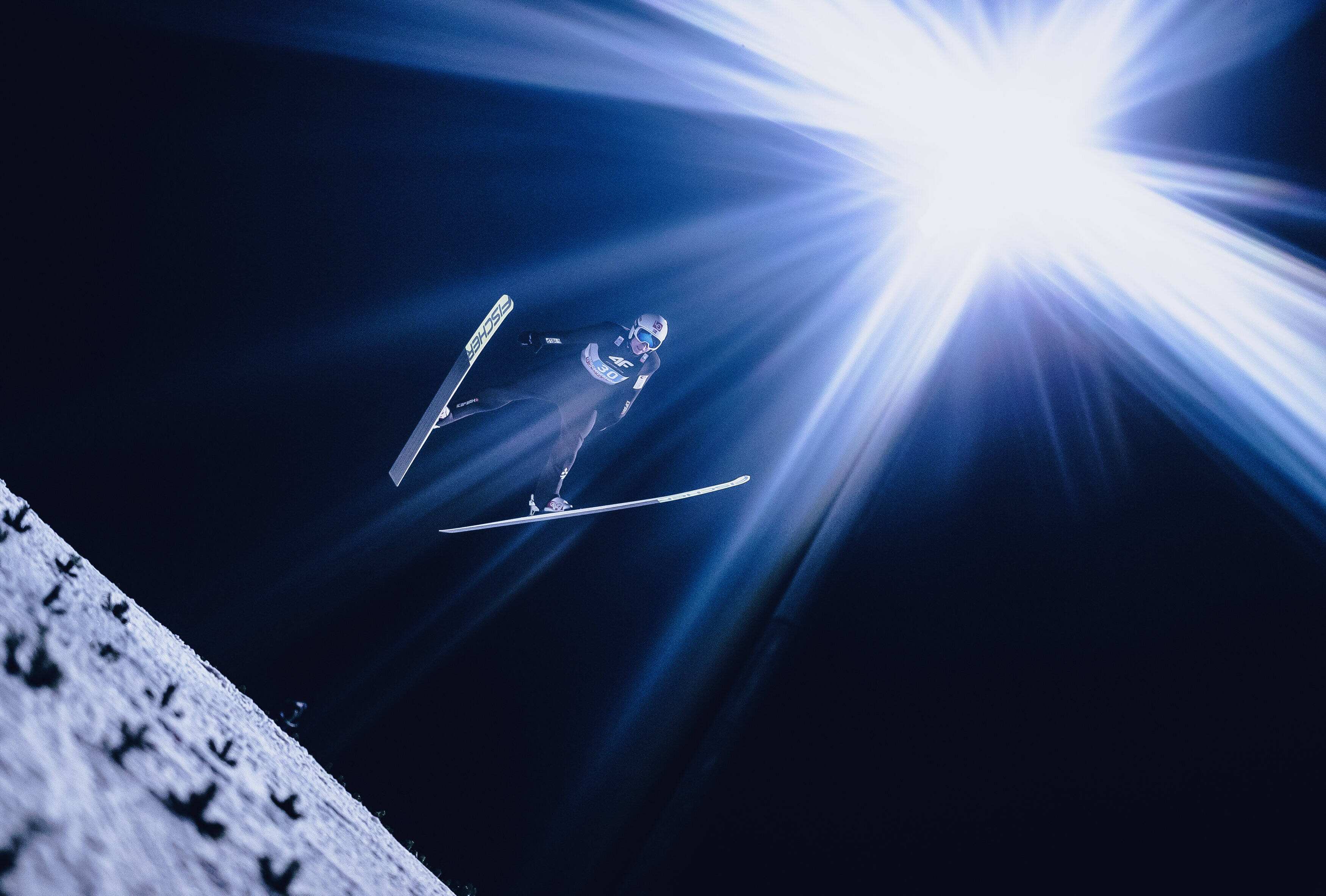In this striking photograph taken from below, we see a ski jumper soaring through the air, captured mid-flight with a dramatic and dynamic perspective. The jumper, clad in a sleek black and white suit that prominently displays a badge with the number 30 and the logo "4F," is framed nearly dead center. His skis are splayed in a characteristic V position, with "Fischer" written in black text on their white tips, while the rest of the skis remain darker in color. A silver helmet and goggles complete his aerodynamic look. The skier is high above the slope, which is located in the bottom left corner of the image, where small black elements protrude from the snowy surface in what appears to be a backward "T" shape. The sky above is a stark black, creating a striking contrast with the bright, star-shaped burst of light emitting multiple rays from just above the jumper's head, possibly from a powerful spotlight. The light casts sharp white and blue glares across the photograph, adding to the ethereal and high-energy atmosphere of the scene.